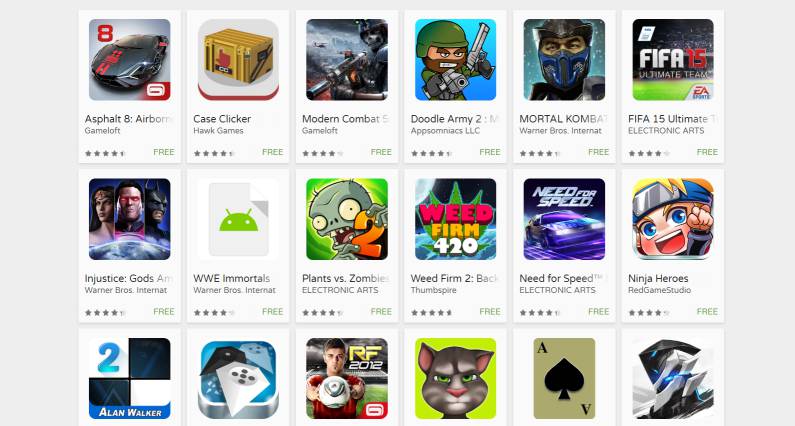This screenshot captures a detailed view of an app store page dedicated to games. The layout is neatly organized into three distinct rows, each showcasing various popular game titles. 

**Top Row:**
1. **Asphalt 8: Airborne** - Developed by Gameloft.
2. **Case Clicker** - Developer details displayed.
3. **Modern Combat 5** - Developer listed.
4. **New Lorimer 2** - Developer specified.
5. **Mortal Combat** - Developer noted.
6. **FIFA 15 Ultimate** - Developer shown.

Each game in the top row features:
- The developer's name beneath the title.
- A star rating system indicating user reviews.
- The price positioned in the bottom right corner.

**Second Row:**
1. **Injustice: Gods Among Us** - Displayed with an illustrative game icon.
2. **WWE Immortals** - Presented with its intriguing cover art.
3. **Plants vs. Zombies** - Recognizable by its iconic game image.
4. **Need for Speed** - Accompanied by engaging game art.
5. **Ninja Heroes** - Identified by its vibrant game icon.

Each game in the second row includes:
- An eye-catching game icon and artwork above the title.
- The developer's name.
- Star ratings to reflect user satisfaction.
- The price in the bottom right corner. 

Together, these rows provide a comprehensive overview of available games, complete with all essential details for potential users.